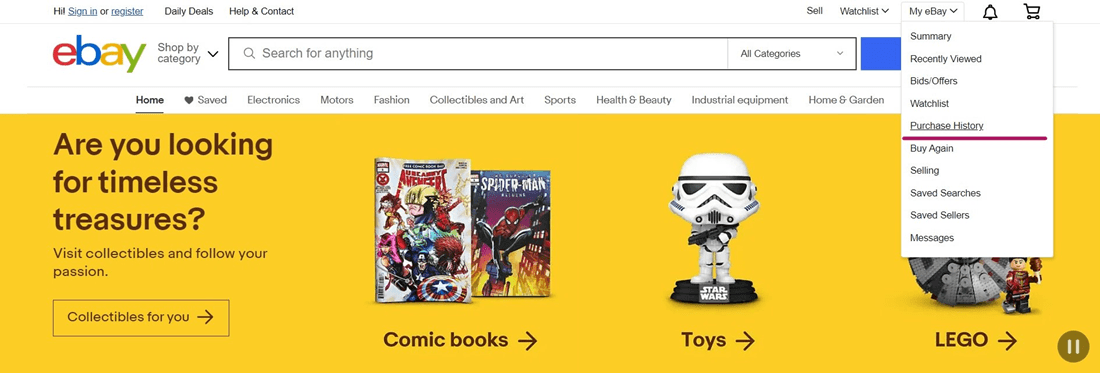Here's a detailed and cleaned-up caption for the described eBay page image:

---

The eBay page features a clean white background. At the upper left corner, black text lists options for "Sign In", "Register", "Daily Deals", and "Help & Contact". Adjacent to these, a blank white space leads to the upper right section where options for "Sell", "Watchlist", and "My eBay" are displayed. 

The "My eBay" dropdown menu includes "Summary", "Recently Viewed", "Bid/Offers", "Watchlist", "Purchase History" (highlighted and underlined for emphasis), "Buy Again", "Selling", "Saved Searches", "Saved Sellers", and "Messages". At the very top, there are icons for notifications, represented by a bell, and a shopping cart.

Centrally, the iconic eBay logo stands out with its signature red, blue, yellow, and green letters. Below the logo, "Shop by Category" and a white search box can be found. The search box, typically featuring a blue arrow for initiating searches, is partially obscured by an overlapping white dropdown menu.

Dominating the main body of the page is a prominent section against a white or light yellow background. Black text on the left invites users to explore "timeless treasures" in the Collectibles category, with a prompt to "visit collectibles and follow your passion." Three clickable sections beneath this invitation highlight Comic Books, Toys, and Lego.

The comic books showcase covers featuring Spider-Man and The Avengers. The Toys section displays an image of a white Stormtrooper figurine. The Lego section suggests a gray Millennium Falcon set with a partially visible Han Solo figurine, though it is partly covered by the intrusive dropdown menu. 

This description concludes as the page signals an end to this segment before moving on to the next one.

---